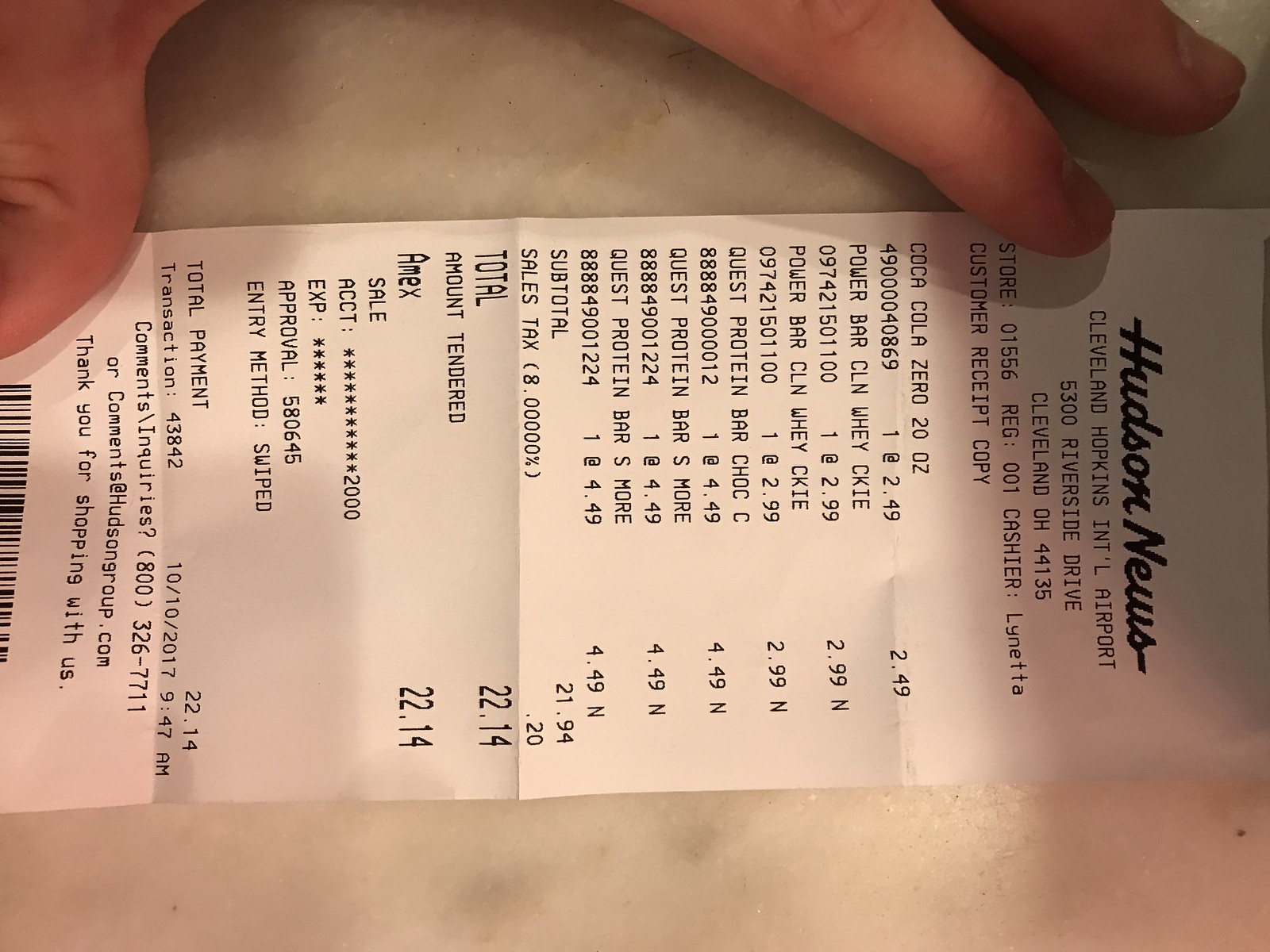In this image, we see a receipt held sideways. The person holding the receipt has their index finger and thumb touching it at the top. The background platform, against which the receipt is held, is white, matching the color of the receipt itself. The print on the receipt is black. At the top of the receipt, the text reads, "Hudson News," followed by "Cleveland-Hopkins International Airport." Below that, the address is listed: "5300 Riverside Drive, Cleveland OH 44135." It includes additional details such as the store number ("Store 01556"), register number ("REG 001"), and the cashier's name, "Lynetta," spelled "L-Y-N-E-T-T-A." The receipt is labeled as a "Customer Receipt" at the bottom.